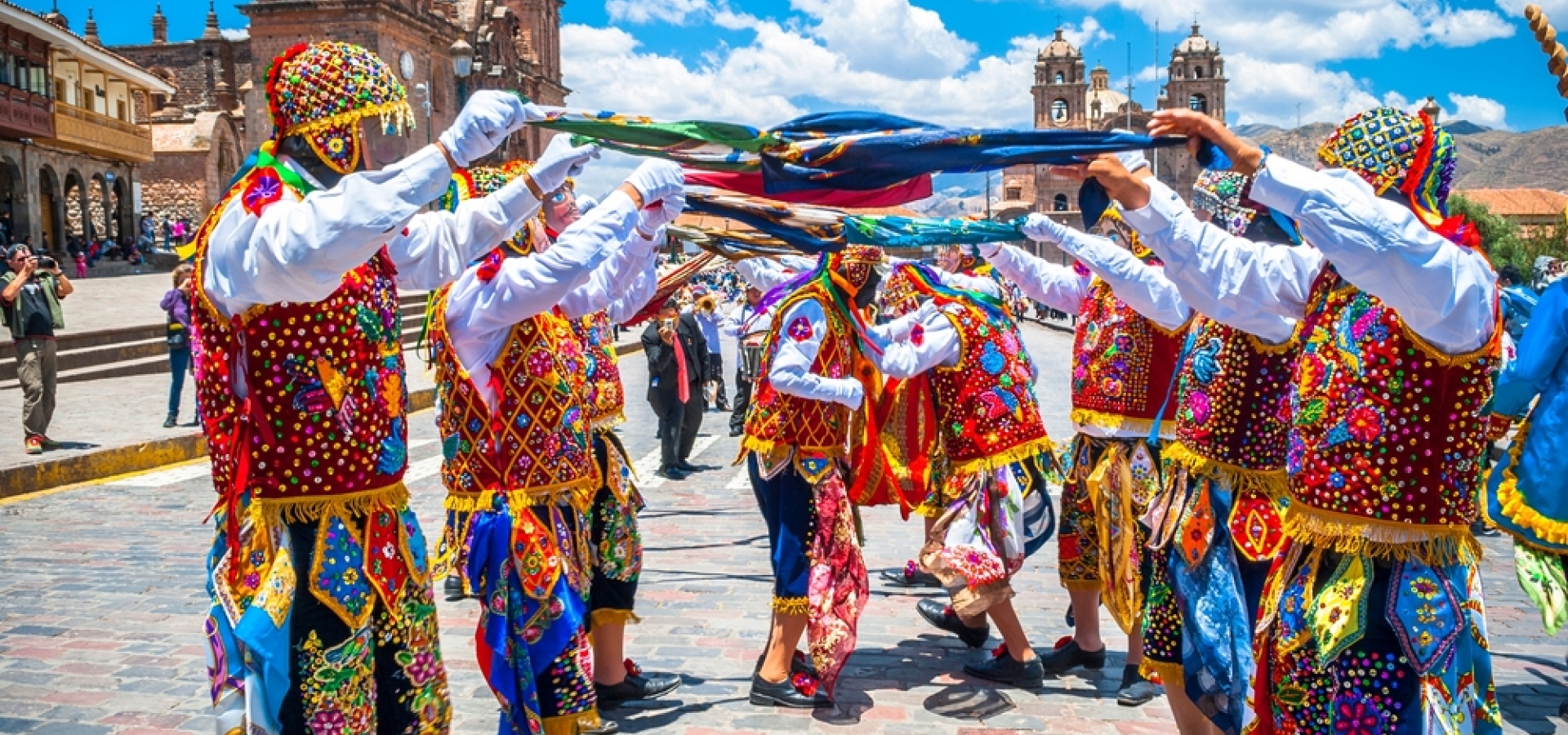In this vibrant outdoor photograph, a row of six individuals, three on each side, are dressed in intricately colorful costumes, standing in a ceremonial formation on a street. Each person is adorned in a multicolored vest with an array of vivid shades including red, blue, orange, yellow, and pink, along with matching pants or skirts. Their outfits are embellished with dots or marbles and complemented by rainbow-colored hats with yellow trim. White button-down shirts and white gloves peek from beneath their festive vests. All the participants appear to be wearing masks, adding to the elaborate nature of their attire.

Between the two rows, which are facing each other, the individuals hold wrapped and bundled flags, raising their arms in what seems to be a synchronized display. Photographers and onlookers are present, capturing the spectacle. In the distance, more people dressed in similarly colorful get-ups can be seen.

The scene is set against a backdrop of historic-looking buildings under a clear blue sky dotted with white clouds. To the right, a mountainous landscape peeks into the frame, further setting the scene possibly in Peru, perhaps during a festival or parade such as the Festival of Cusco, although the exact event remains unspecified.